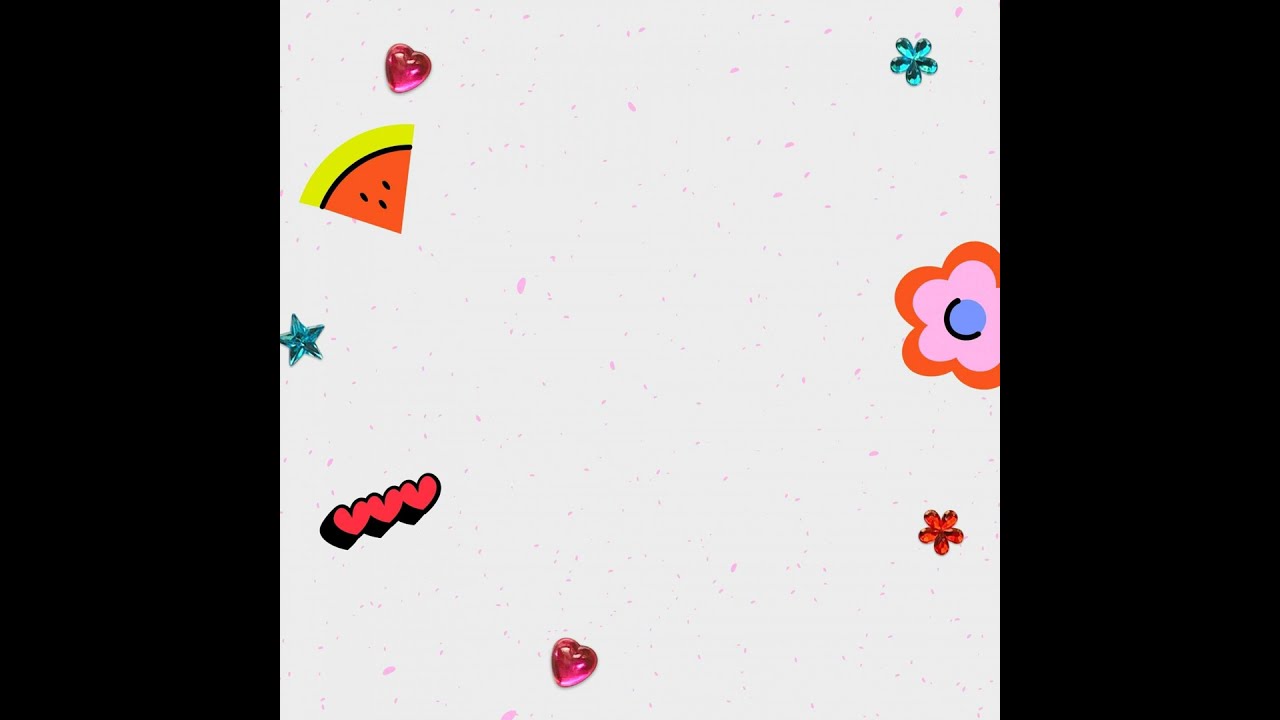The image is a detailed digital collage set against an off-white background, speckled with faint pink and tiny royal blue sparkles. Central to the design is a vibrant slice of watermelon, featuring distinct layers of yellow, orange, and a black-edged border, with three seeds in its center. Directly beneath the watermelon slice is a green and blue star, followed by a deep red shiny heart positioned below the star. Further down are three interconnected red hearts leading towards the bottom middle, where another tilted red heart lies. 

On the right edge of the image, there are vividly colored flowers, including an aqua green five-petaled flower, and a larger flower with a red border, pink center, and a blue button-like core. Below these is a five-petaled maroon red flower. The entire composition is framed by large vertical black strips on both the left and right edges. The playful and colorful elements scattered throughout the center evoke the feel of children’s drawings, creating a whimsical and engaging visual.